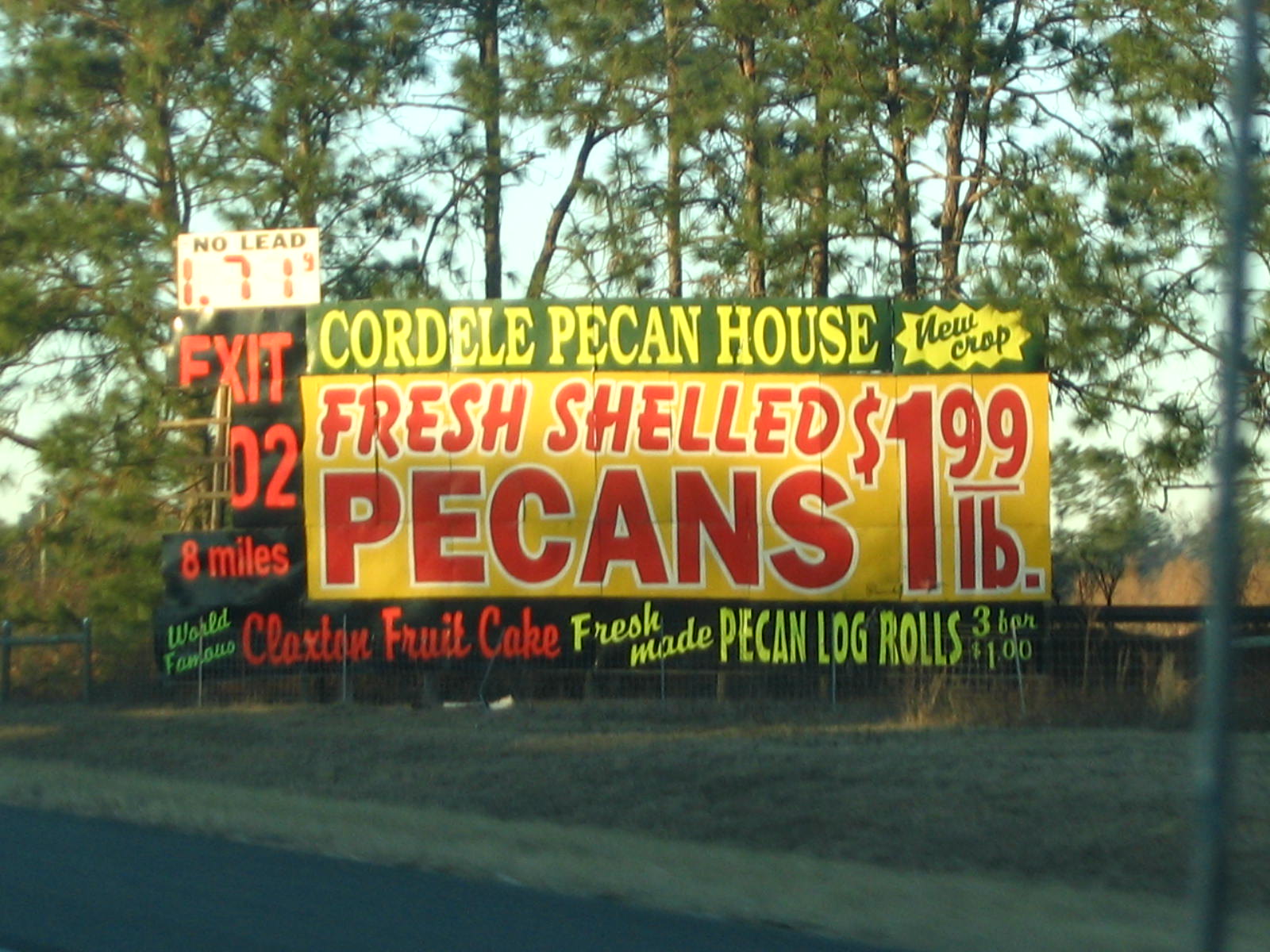A large, vintage, non-digital billboard is prominently displayed amidst a cluster of pine trees, suggesting it's located in East Texas along a highway. The sign is weathered, with a broken fragment lending it an even older appearance. In the background, a fence can be faintly seen through the trees. The primary advertisement on the billboard reads "Cordell Pecan House" in bold yellow lettering on a green backdrop. The central message boasts "Fresh Shelled Pecans" for $1.99 per pound, while on the left side, a notation indicates "NOLAD gas price" at $1.71 per gallon, hinting at the image's age given current gas prices. Below, the sign directs travelers to exit 028 miles ahead. The bottom of the billboard touts "World Famous Claxton Fruitcake" and "Fresh Made Pecan Rolls" priced at just $3.00, further reinforcing the historical context with surprisingly low prices.